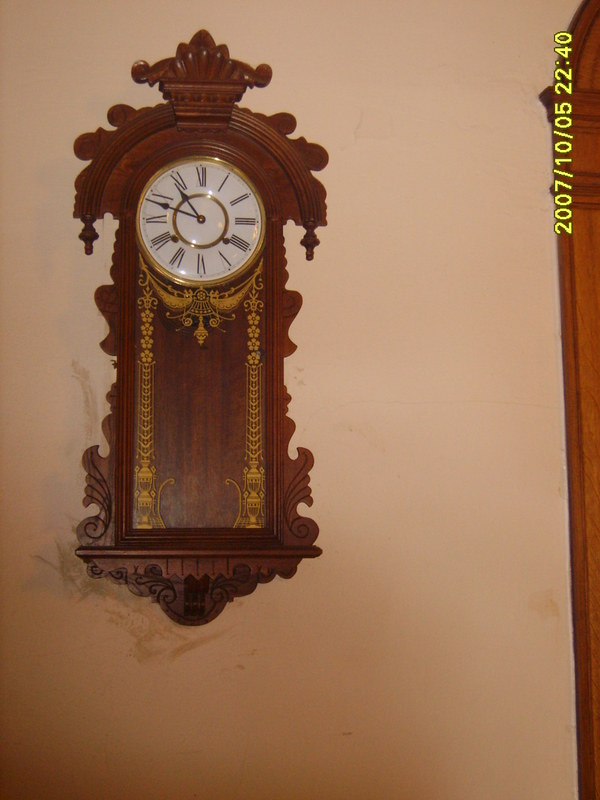This image depicts an ornate wall clock that closely resembles a grandfather clock, albeit without a pendulum. The clock is mounted on a beige-colored wall, which shows signs of wear and marring, suggesting that the clock has been moved over time. A wooden door frame can be seen on the right-hand side of the image. The clock itself is crafted from deep brown wood and features intricate detailing. The clock face is white, displaying the time at approximately 10:48 or 10:49 with black hands and Roman numerals, and is surrounded by a gold outline. Below the clock face, a rectangular section adorned with gold detailing includes four floral designs and tall columns on each side. The photograph is time-stamped in yellow ink with the date October 5th, 2007, at 22:40.